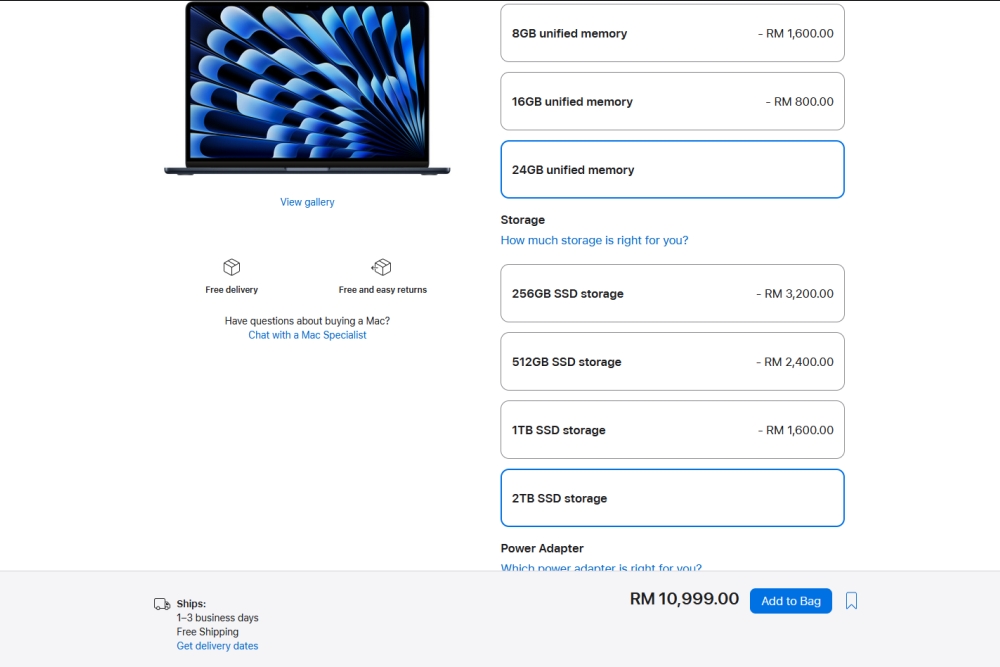The image displays a section of a website where a user is in the process of configuring a customized Mac laptop. On the left side of the screen, there is a picture of the laptop, with an option to view the gallery highlighted in blue beneath it. Below the gallery option, text indicates "Free Delivery" in dark gray, accompanied by an icon. Next to this, there is another icon with the text "Free and Easy Returns" below it. Further down, centrally aligned and also in dark gray, is the question "Questions about buying a Mac?" with an actionable blue link beneath it stating "Chat with a Mac specialist."

On the right side, various configuration options are displayed. The first set of options pertains to memory, showing choices for 8GB (RM800) and 16GB (RM1600) of unified memory, with the selected option being 24GB. Below the memory selections, the available storage options are detailed. Choices include 256GB SSD (RM3200), 512GB SSD (RM2400), and 1TB SSD (RM1600), though there is a noted discrepancy here. The user has selected the 2TB SSD storage option, which isn't fully visible. The cumulative cost of the selected configuration is displayed as just under RM11,000, with an actionable button to add the customized Mac to their shopping bag, as the website uses "bag" instead of "cart."